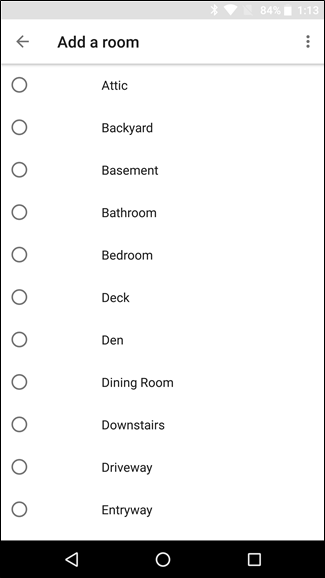The image depicts a list created on a smartphone. At the top, there's a gray notification bar showing a Wi-Fi icon, a battery at 84%, and the time 1:13. Below the notification bar, there is a heading titled "Add a room," accompanied by a left-pointing arrow on the left side and three vertical dots followed by a vertical line on the right side. Below this heading is the actual list, which features various room names. Each room name is preceded by an empty circle, indicating they can be selected or filled in. The listed rooms include: Attic, Backyard, Basement, Bathroom, Bedroom, Deck, Den, Dining Room, Downstairs, Driveway, and Entry. All circles next to the room names are currently unfilled, merely outlined.

At the bottom of the screen, there's a black border containing three outlined icons in white. Positioned on the left is a left-pointing triangle, in the center is a circle, and on the right is a square. The list and the interface appear clean and straightforward, with no additional images or graphical elements aside from the text and icons.